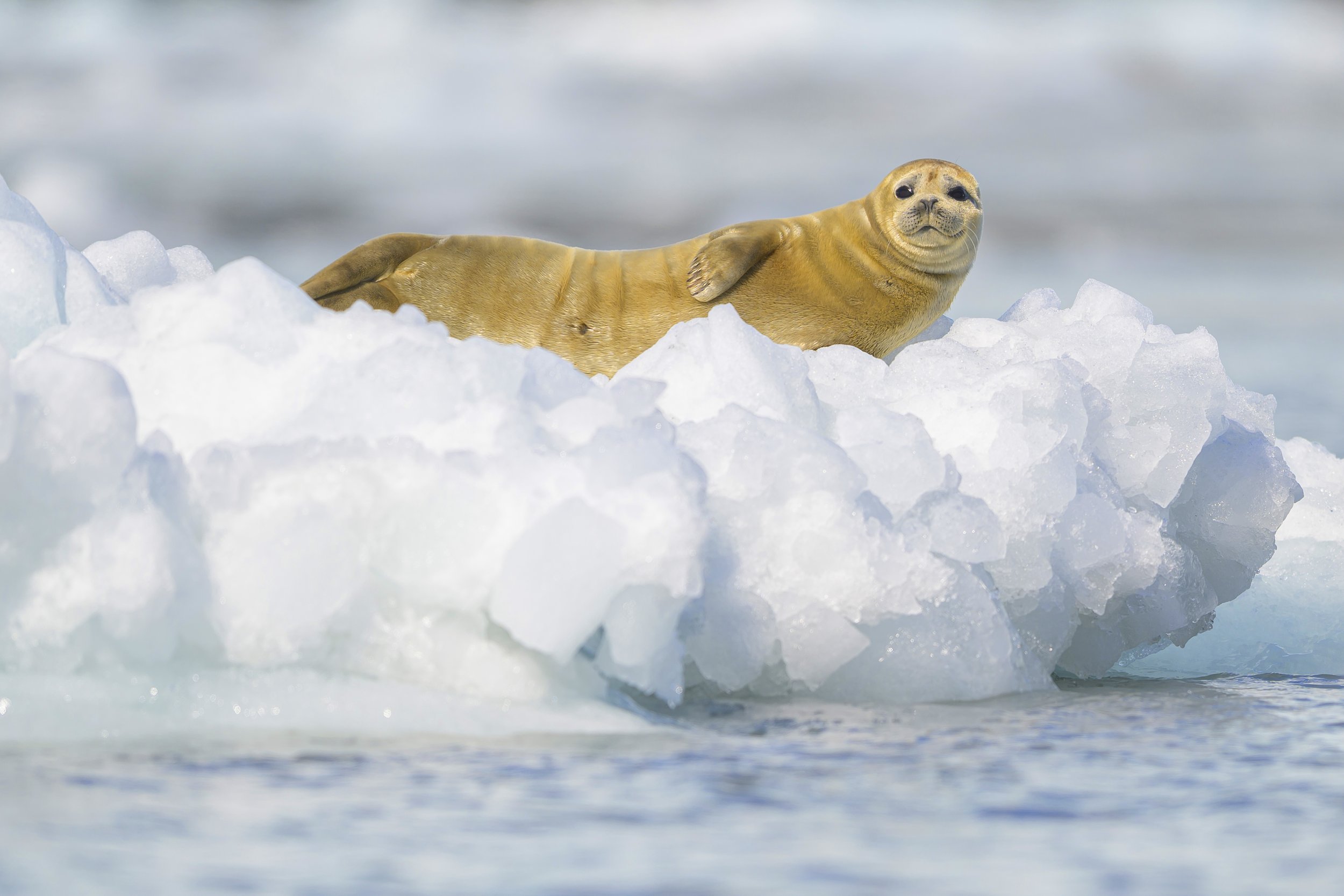This image captures a young sea otter lounging on a large, jagged chunk of ice that resembles a natural sofa. The otter's coat features a unique mix of brownish-white to yellowish-brown hues, with a lightly colored belly. Its position is relaxed yet attentive, as it gazes curiously at the photographer, appearing slightly disturbed by the attention. The otter's flippers are visible, with one positioned in front and the others tucked beneath its body. The ice beneath the otter forms an intriguing pattern of jutting chunks, highlighted by a bluish tinge from the frozen water below. Surrounding the scene is a blurred backdrop, characterized by gray and white clouds, which focuses all attention on the otter and its icy resting place. The overall impression is one of serene beauty amidst the cold and stark environment.